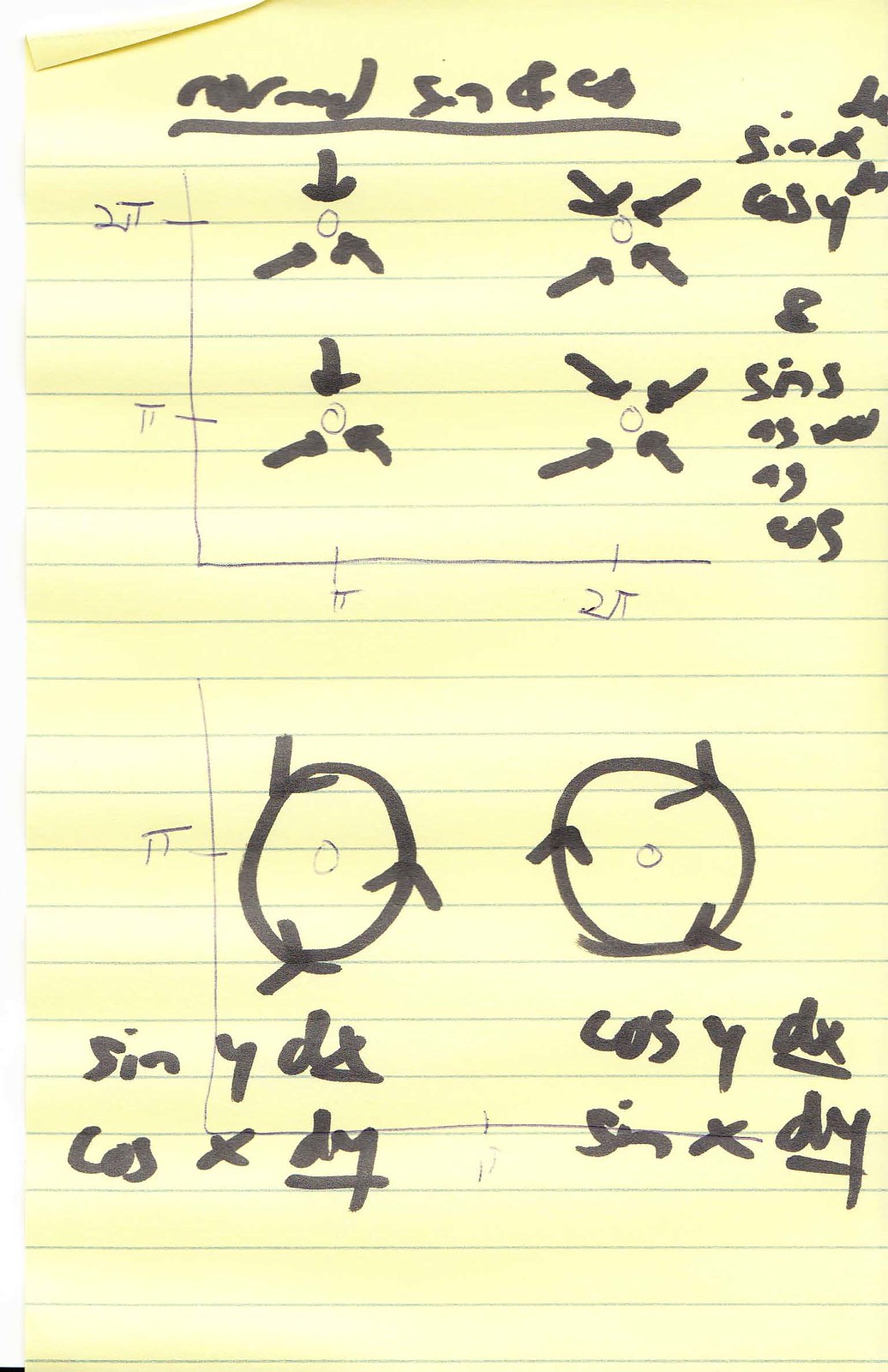In this image, you see a yellow piece of writing paper with subtle bluish-purple lines. Various markings are scattered across the paper; there's black marker, along with what appears to be ink or pen writings.

At the top of the image, written in ink, is a numeral "2" accompanied by a "T" symbol positioned slightly to the side. Below these characters, there is an incomplete square: a single vertical ink line and a horizontal line forming an inverted "L". Extending from this horizontal line, multiple small lines intersect perpendicularly, possibly resembling a basic diagram or chart.

Near these lines, several small circles and three black marker arrows point toward one of the circles. There are four instances of arrows pointing to circles in the upper part of the image. On the right-hand side, some writing is visible, though its content is not entirely clear in the description. 

At the bottom of the paper, there are two large black ink circles, distinct and prominent, standing out from the other markings above. The entire image captures a mix of hurried sketches and precise markings, creating a visually intriguing composition on the yellow lined background.